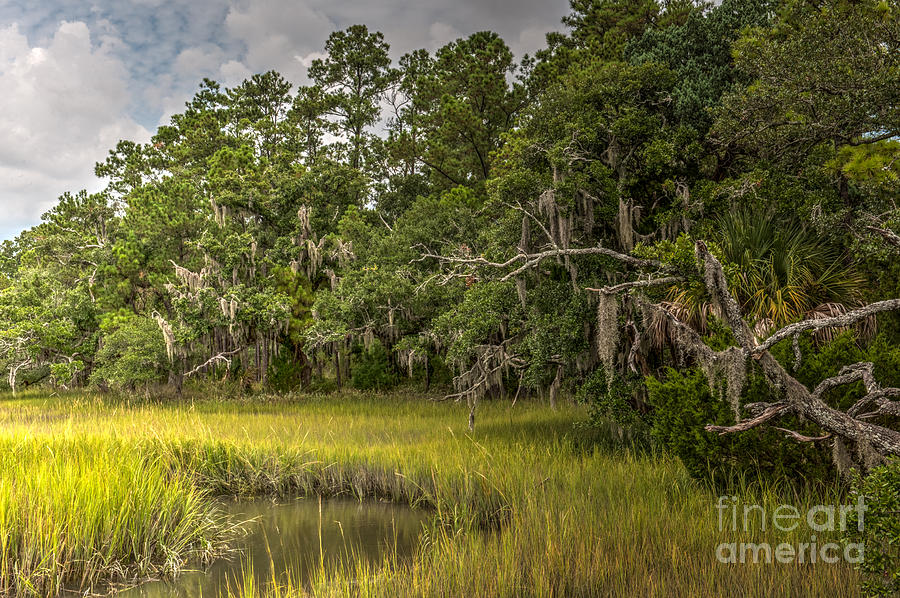This outdoor scene captures a tranquil wilderness area characterized by its lush vegetation and a sense of isolation. Dominating the bottom of the image is an open grass field interspersed with green and yellow hues, which reflect the sunlight. In the bottom left corner, a small, murky body of water adds to the marshy ambiance of the scene. The midsection of the image, extending to the upper right, is filled with dense old-growth trees, some adorned with gray moss hanging down almost to the marsh level, reminiscent of the landscapes seen in Southern Louisiana. The upper left of the image features a sky filled with fluffy white clouds against a blue backdrop, indicating an impending thundershower with sunlight reflecting off the clouds. Scattered throughout are logs and branches in shades of brown and whitish, adding texture to the scene. The bottom right corner is marked with a watermark that reads "Fine Art America" in gray letters. This photo beautifully captures the natural, swampy wilderness, devoid of human presence, and showcases a harmonious blend of blue, gray, white, green, light green, brown, and yellow colors.